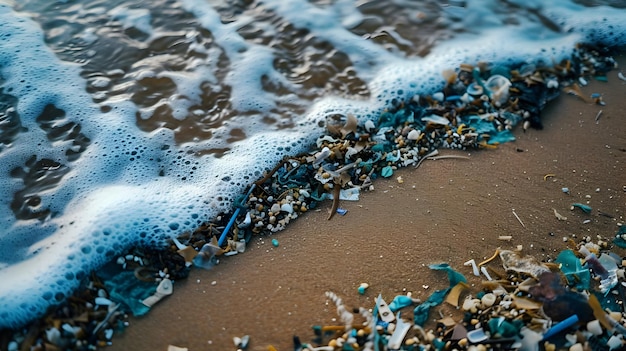A disheartening scene unfolds in this beach photograph, where the sandy shore, a wet brown hue, meets the clear ocean waters. As the gentle waves advance, the edge of the water is marked by a stark collage of debris: a blue straw, assorted pieces of plastic, small broken shells, and various other types of trash litter the area where the sea and sand converge. White foam from the surf contrasts sharply with the pollution it washes over. In the lower right corner of the image, a small, concentrated pile of garbage further mars the natural beauty of the beach. Though the individual pieces of debris are minute, their collective presence dominates the scene, painting a poignant picture of environmental neglect.